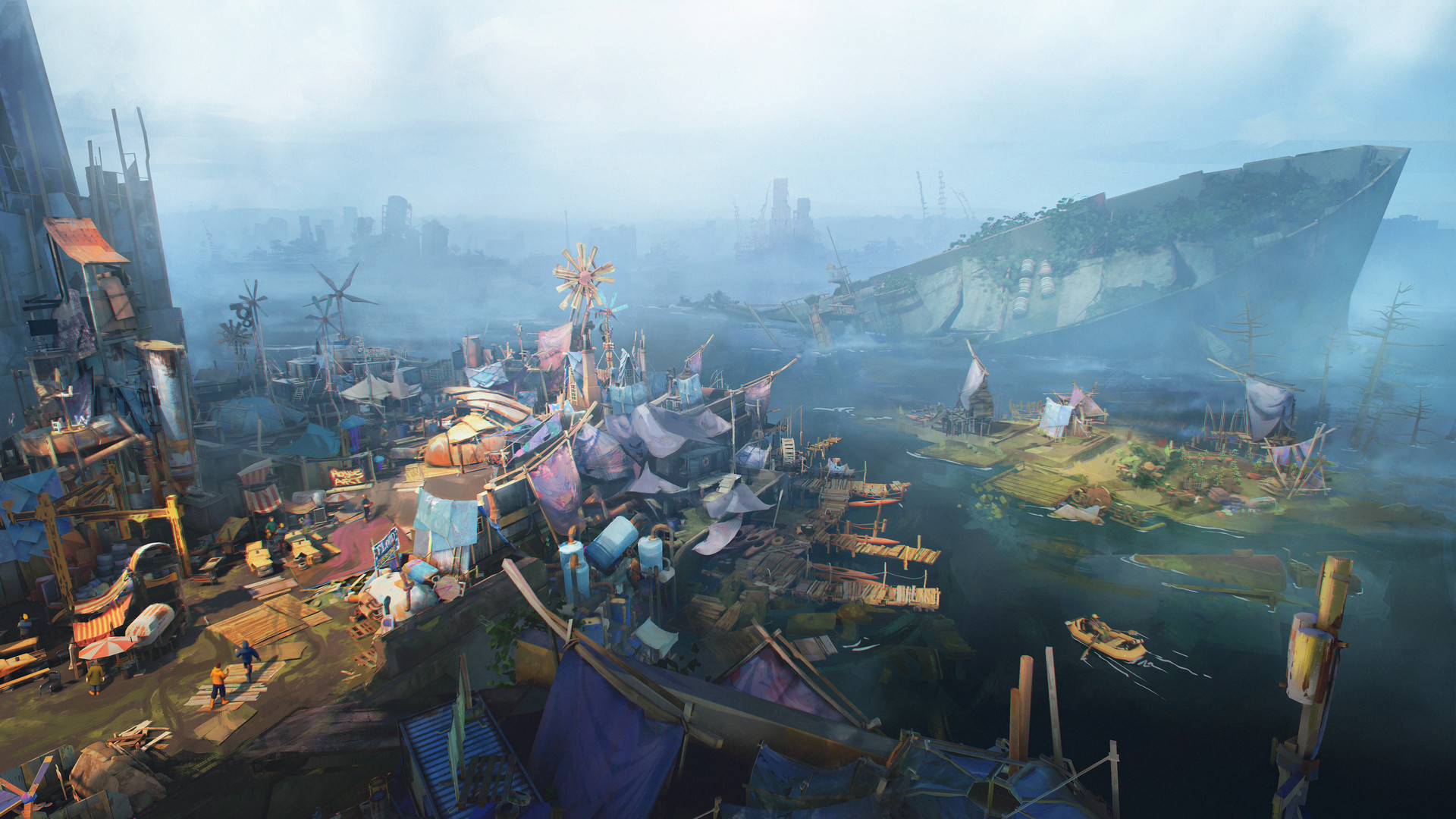The image is a highly detailed and impactful artwork depicting a catastrophic shipwreck near the shore. The bow of the ship is still visible above the water, while the stern has already submerged. The surrounding water and sky are shrouded in thick fog, suggesting a sense of mystery and desolation, with possible hints of a distant city or additional ships obscured by the haze.

In the foreground, there is a chaotic scene filled with debris and makeshift arrangements. Clotheslines and various textiles, likely salvaged from the ship, are laid out to dry, giving the impression of a desperate attempt to salvage usable items. Various belongings, resembling what you might find in a house, are scattered around, adding to the sense of disorder. Amongst this mess, a small windmill stands, and rafts appear to be used for transporting or storing the rescued goods.

Off to the side, there is a cluster of makeshift huts, suggesting that people have begun to form a community out of the wreckage, perhaps as a result of a dystopian future or a catastrophic event. The scene is predominantly rendered in grim grays and blues, except for this community area where splashes of pink, purple, and blue bring a fleeting sense of life and hope. Vines growing over some parts of what appears to be a large yacht or shipping container highlight the passage of time and nature reclaiming the scene. The overall atmosphere is one of poignant desolation yet hints at human resilience in the face of disaster.